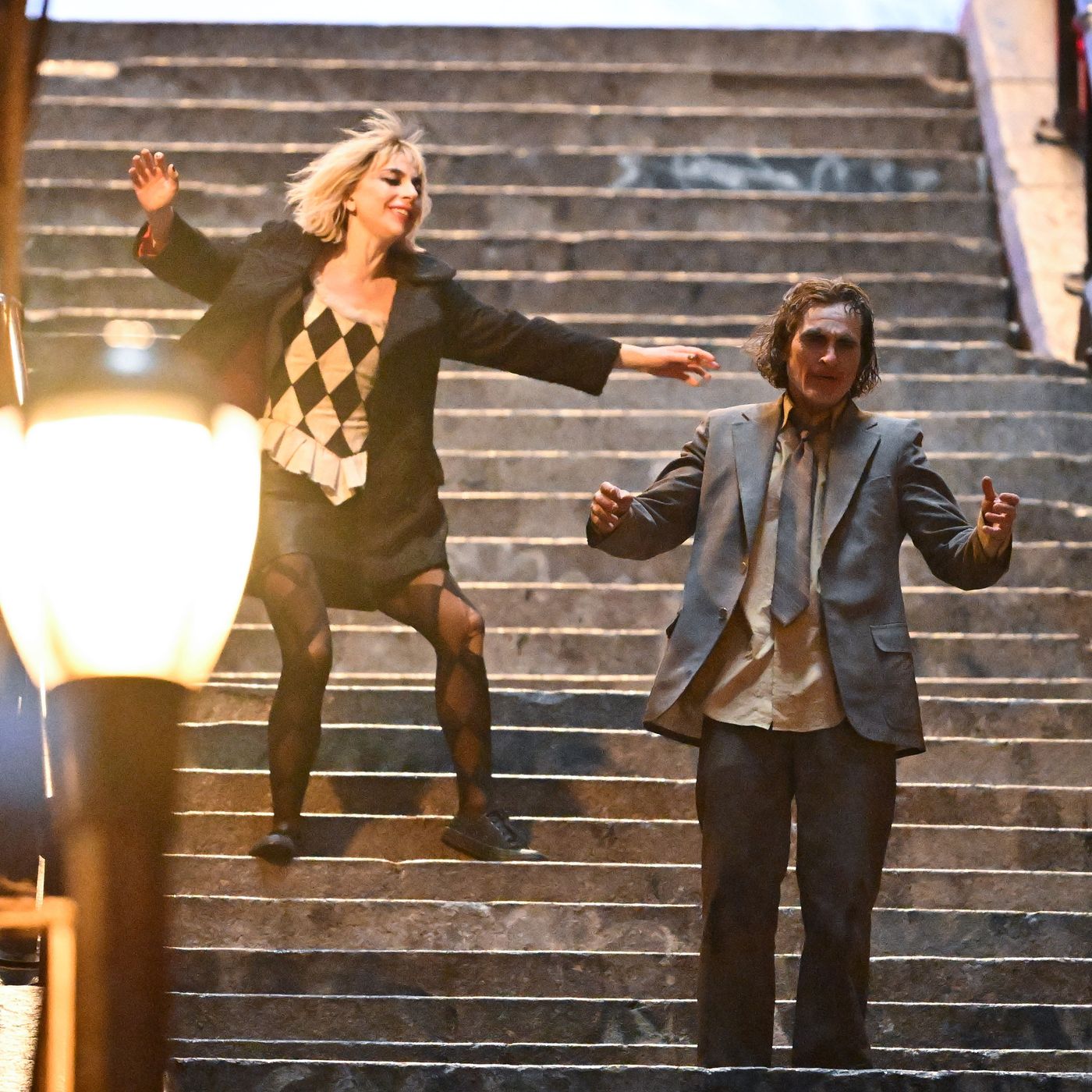The image captures a cinematic scene on a flight of concrete stairs, likely from a practice or production still of a film resembling "The Joker." On the right, a man stands slightly lower on the steps, wearing an unbuttoned gray business coat over a yellow button-up shirt with a loose brown tie, paired with dark brown pants. His long, messy hair complements his distraught expression as he stretches his arms forward. On a higher step, the woman to his left is dynamically posed with slightly bent knees and outstretched arms, as if in mid-dance or landing. She has short brown hair adorned with gold hoop earrings and wears a short black dress with a checkered top featuring white frills at the bottom, black stockings, and black tennis shoes. Her attire is completed by a black business coat with a red liner. A bright yellow lamp post is prominently visible at the bottom left, adding to the scene's dramatic ambiance.